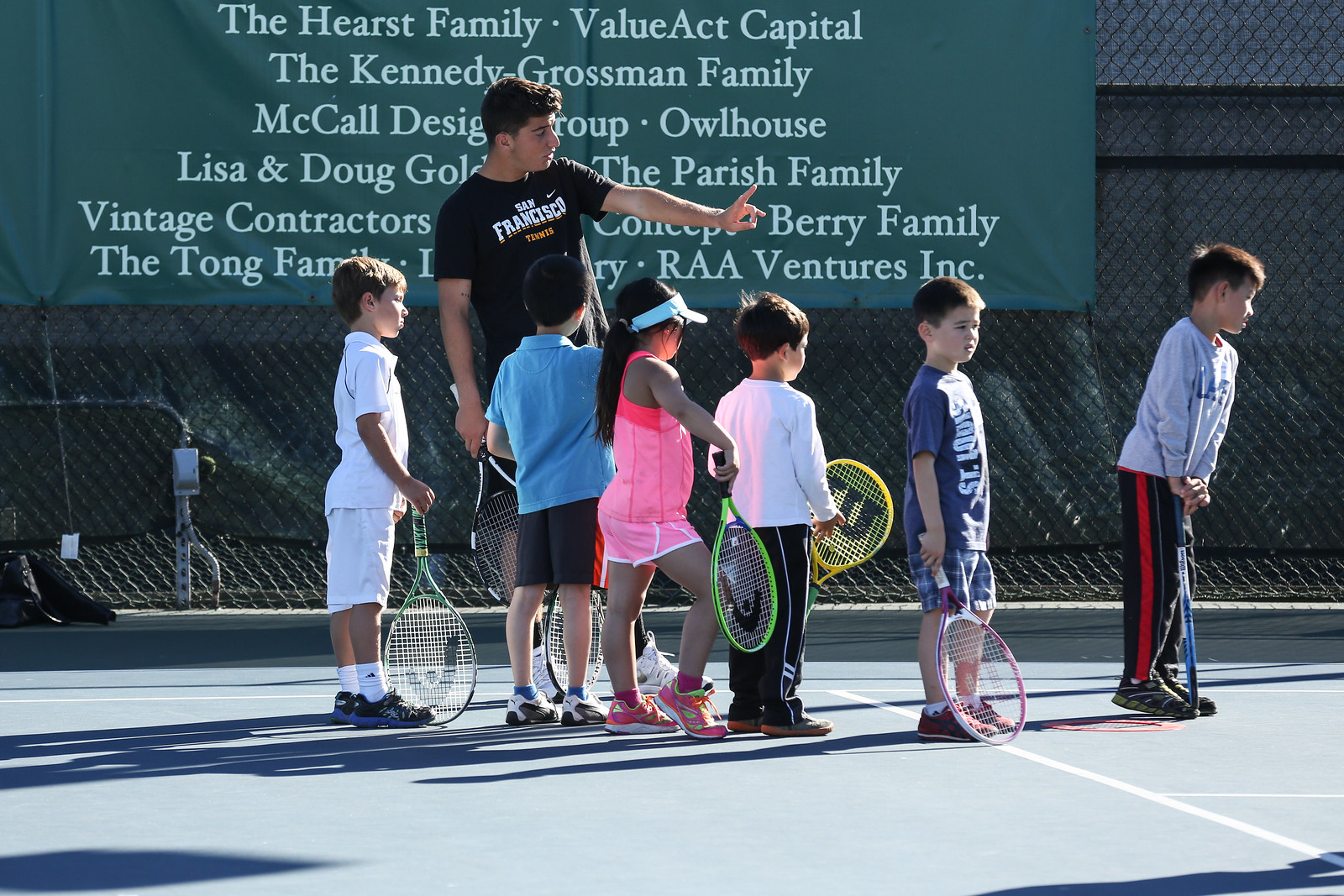This photograph captures a vibrant scene on a tennis court featuring six young children and their instructor. The children, comprised of five boys and one girl, are dressed in sports gear and each hold a tennis racket. An adult male instructor, clad in a black shirt and also holding a racket, appears to be speaking and pointing off-camera, capturing the children's attention. Enclosing the court is cyclone fencing adorned with a green banner showcasing numerous sponsors such as the Hearst family, Value Act Capital, the Kennedy Grossman family, McCall Design Group, Owl House, Lisa and Doug Gold something, the Parrish family, Vintage Contractors, Concept Berry family, the Tong family, and RAA Ventures Inc., among others that are partially obscured. Shadows cast across the court add depth to the lively atmosphere of this instructional moment.